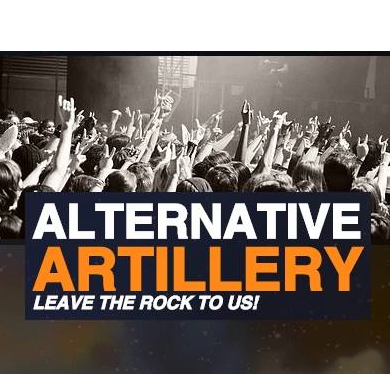The image captures a dynamic, black-and-white concert scene filled with smoke and energetic concert-goers. At the heart of the image, a crowd of potentially hundreds of people, mostly young to middle-aged, can be seen raising their arms and forming V symbols with their fingers, enraptured by the performance on stage. A hazy, smoke-laden atmosphere envelops the scene, focusing attention on a distant guitarist performing on stage, partially obscured by the smokiness. Above the stage, a window with blinds is visible, splitting the background into two sections. Prominently in the foreground, layered white and orange text reads, "alternative artillery, leave the rock to us!" The phrase "alternative artillery" is displayed in white and orange lettering respectively, followed by "leave the rock to us!" in smaller white text, encapsulating the concert's energetic and rebellious spirit.